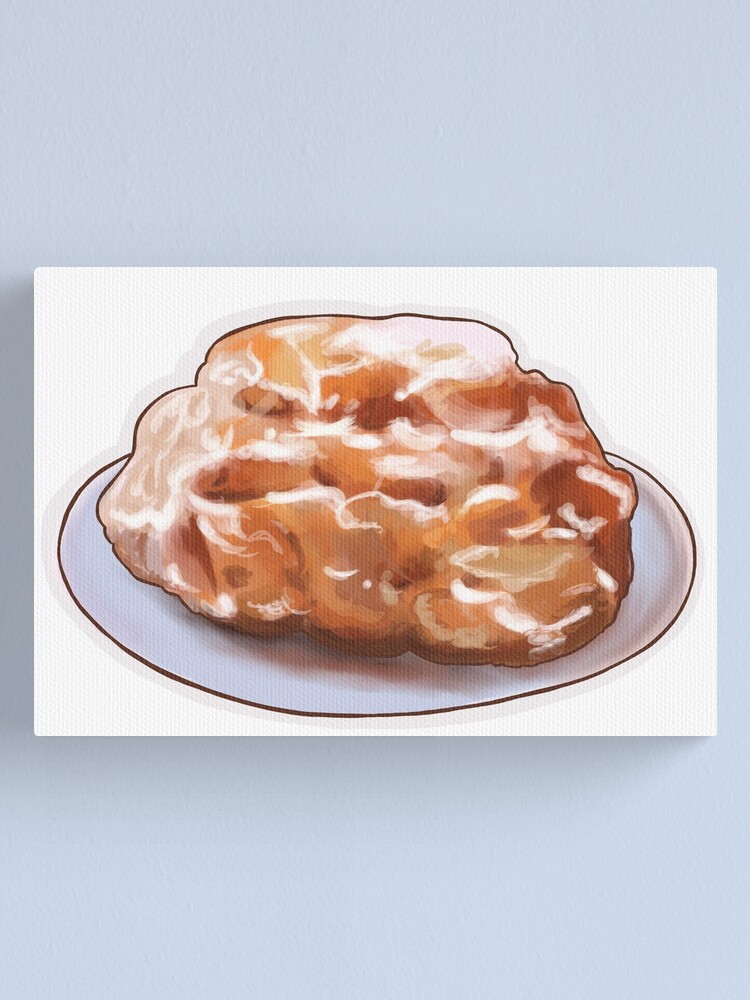The image depicts a rectangular canvas mounted on a light blue wall. The canvas features what appears to be a digitally rendered painting or photographic artwork of an ambiguous food item. The food item is brown, lumpy, and circular, resembling an old-fashioned donut or a pastry with an irregular shape and a shiny, glazed appearance. It is set on a plate with a bluish tint. The artwork is outlined in black and uses a mix of colors, including brown, red, cream, and orange, lending it an abstract and somewhat unclear visual. The background of the canvas itself is a stark white, helping the colors of the subject stand out, but no text is present to provide additional context or clarity. The overall impression is of an art piece that attempts to depict a pastry in a stylistic manner, giving an impression of a product page for canvas art.